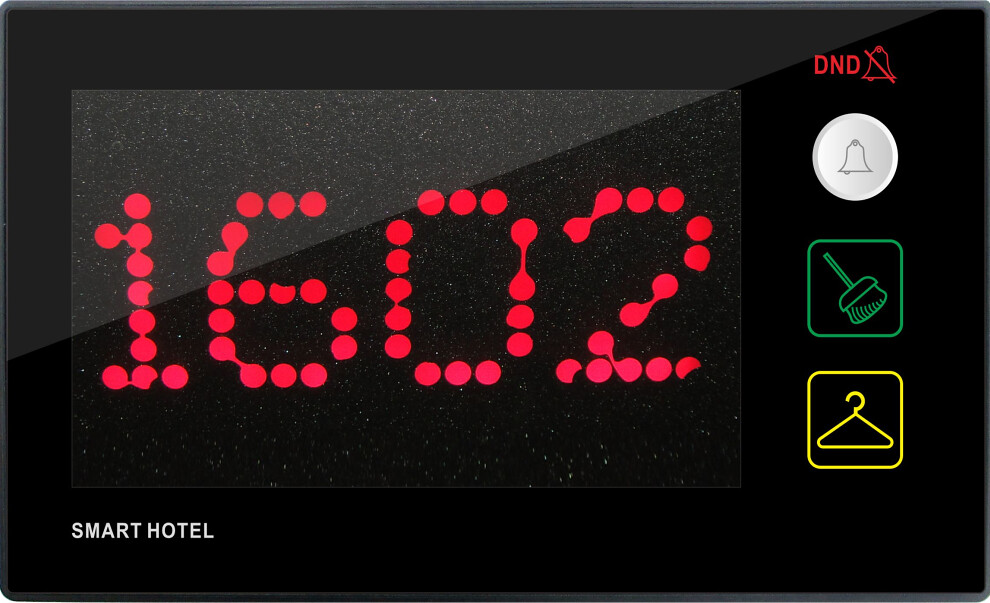The image shows a sleek, rectangular, hotel device with a glossy black and gray background. The central digital display, formed in red dots, reads "1602." Below this, the words "Smart Hotel" are written in white. On the right side, "DND" (Do Not Disturb) is displayed in red with a bell icon crossed out. Beneath these, there is a series of buttons: a white circular button with a bell icon, a green square button featuring a broom, and a yellow square button with a hanger icon. This detailed interface likely allows hotel guests to toggle room settings such as do not disturb, request cleaning services, and indicate laundry or dry cleaning needs.